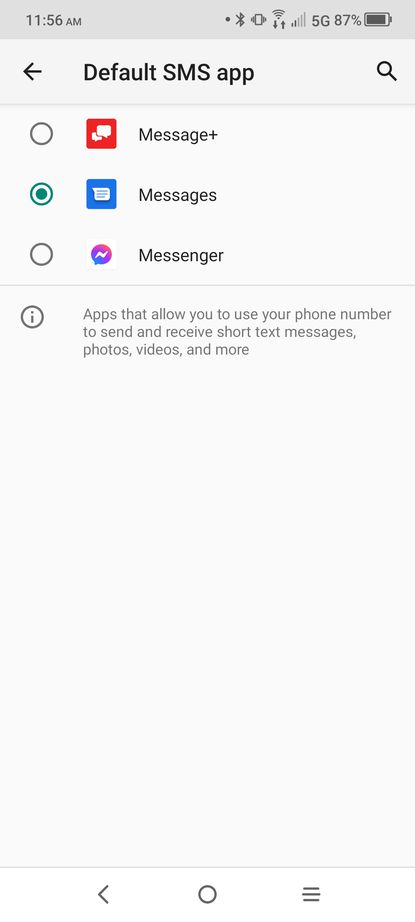Displayed on a user's smartphone screen, this interface features a light gray background with a darker gray status bar at the top. In the top left corner, the time is shown as "11:56 a.m." in dark gray text. To the right of the time are various status icons, including a battery icon indicating a charge level of 87%.

Below the status bar, on a pale gray background, bold black text displays the heading "Default SMS App", flanked by a back arrow on the left and a magnifying glass icon on the right. Under this heading, a vertical list presents three options: Message Plus, Messages, and Messenger, each accompanied by an icon. The option "Messages" is currently selected, signified by a green-filled circle next to it.

A thin, pale gray line separates the list from additional information below. Beneath this line, an exclamation point enclosed in a gray circle is followed by a light gray text description: "Apps that allow you to use your phone number to send and receive short text messages, photos, videos, and more."